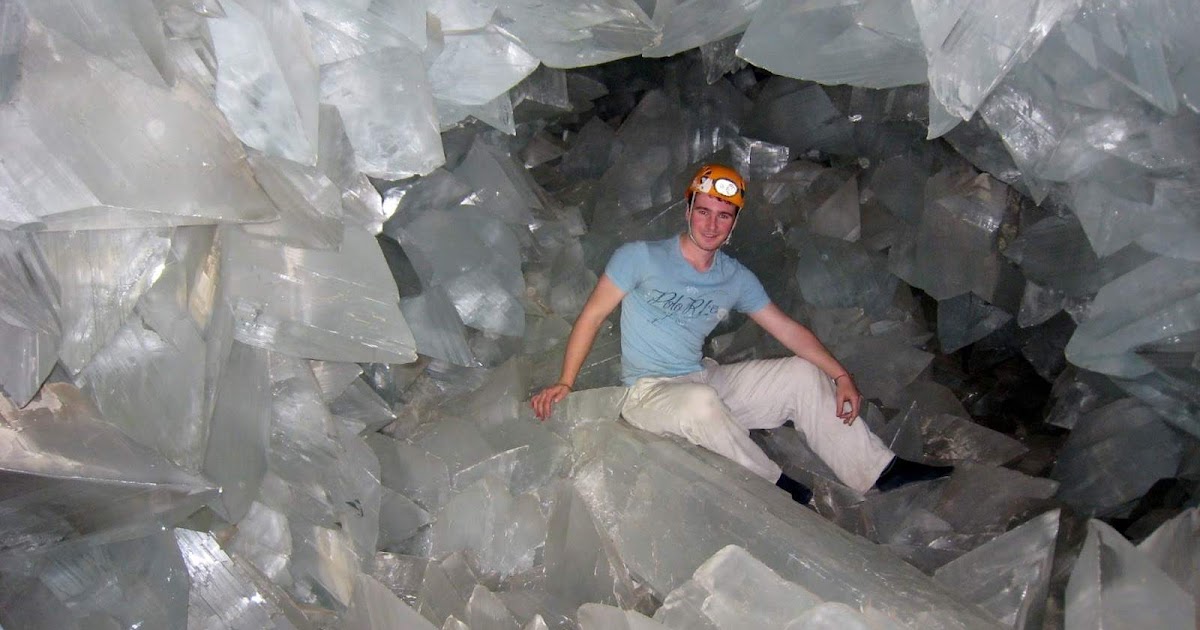In this captivating photograph, a young man is seen sitting comfortably amidst a spectacular ice cave, surrounded by thick, jagged ice crystals. He is dressed in a light blue short-sleeved t-shirt adorned with a blue print on the front, tan pants, and black climbing shoes. An orange helmet with a flashlight and goggles completes his attire, ensuring both safety and visibility within the cavern. The man is smiling warmly at the camera, his left arm resting casually on his knee while his right hand touches one of the nearby ice crystals. The cave resembles the interior of a geode, with the clear, translucent ice formations creating a mesmerizing backdrop. The man appears to be seated on a significant, sturdy crystal, with the surrounding formations protruding sharply in various directions, enhancing the enchanting and ethereal quality of the scene.